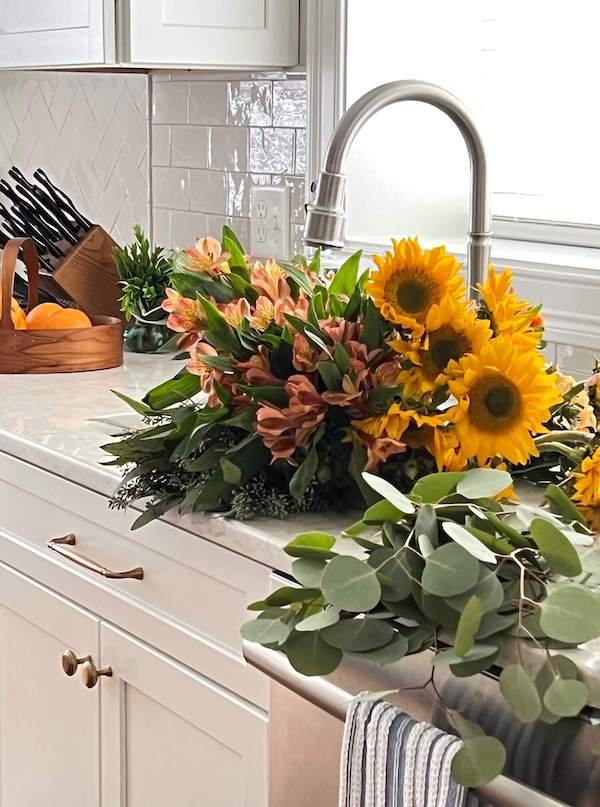This image features a bright, modern kitchen centered around a stainless steel, J-shaped faucet that curves gracefully downward. This faucet is set above a sink brimming with a lush bouquet of sunflowers and pinkish-hued roses, surrounded by an abundance of green leaves. A few stray sunflowers and green leaves rest on the pristine, whitish-gray quartz or marble countertop. The backdrop consists of a glossy white tiled backsplash that subtly shifts in design towards the left side, complemented by upper white cabinets.

Behind the sink, a window framed with white-painted wood and a gray sill lets in plenty of light, enhancing the kitchen's airy feel. To the right, a set of black-handled knives is neatly housed in a light brown wooden knife block. On the counter beside the sink, a round wooden basket brims with fresh oranges.

The lower cabinets are white with gold handles, perfectly matching the drawer and cabinet doors beneath the sink. Adjacent to the sink stands a stainless steel dishwasher, adorned with a blue and white striped dish towel draped over its handle, providing a touch of rustic charm to this clean, contemporary space.